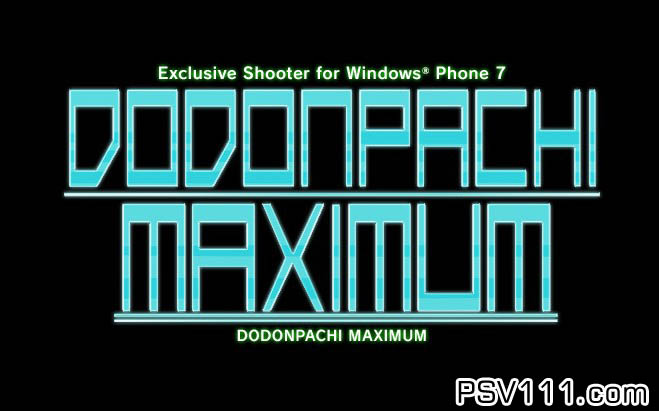The promotional image for a Windows phone features a striking design against a solid black background. Dominating the center, the title "Dodonpachi Maximum" is prominently displayed in a bold, 80s-inspired typographic font reminiscent of the Tron film, with large, creative blue lettering divided into two lines. Just above this, in vibrant yellow-green text, it reads "Exclusive Shooter for Windows Phone 7," emphasizing the exclusive nature of the game. Below the main title, the words "Dodonpachi Maximum" are repeated in smaller green text, reinforcing the game's branding. On the bottom right corner, the URL "PSV111.com" is clearly visible in white outlined letters, each featuring a thin black line, adding a modern touch to the overall retro-futuristic aesthetic of the image. The combination of color typography and illustration underscores the promotional effort, making it a visually engaging advertisement for the Windows phone exclusive shooter.